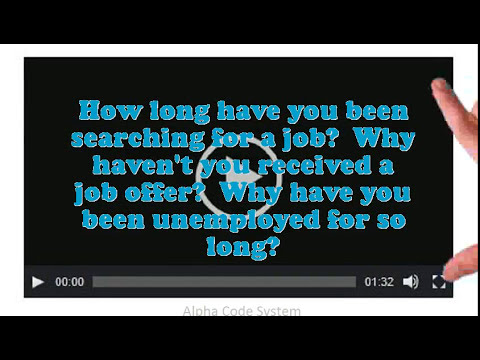The image is a detailed still from a video or possibly a slide showing a paused video with a typical video player interface. The center of the screen prominently displays an arrow indicating play, framed by a black border that suggests a letterbox format. The video's duration is 1 minute and 32 seconds, with the time bar positioned at 0 seconds. Key playback features such as a play button, volume control, and screen expansion option are prominently visible. The scene has a stark white background, interrupted on the right by a partial view of a human hand, specifically the thumb and index finger, as if poised to interact with the screen. The blue, bold text overlaid on the video reads: "How long have you been searching for a job? Why haven't you received a job offer? Why have you been unemployed for so long?" Below this text, in a more subdued gray font, the words "Alpha Code System" appear.